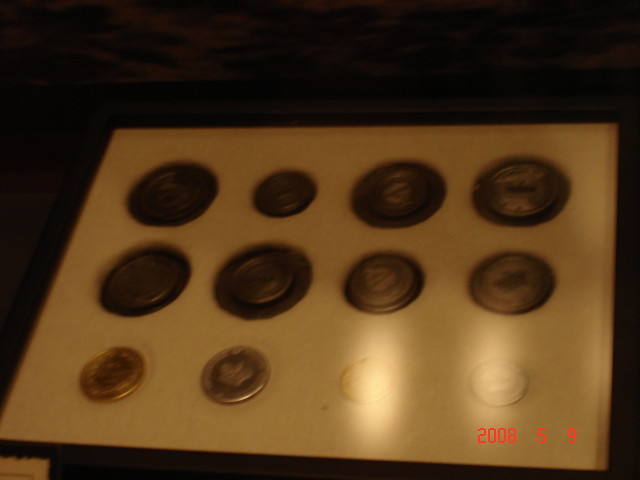The image is a photograph featuring a meticulously arranged display of coins, set against a rectangular, brownish background that gives the photograph a somewhat vintage feel despite its modern date, 2008-05-09, printed in red at the bottom right corner. The coins are housed in a display case, often used for collectible coins like those from the US Mint. There are three rows in the case: the top row features a mix of large and small coins, the middle row contains predominantly large coins, and the bottom row showcases the smallest coins, akin to everyday currency. A distinctive aspect of the display is that it includes both conventional and unusually large, decorative coins, some of which are rotated artistically. The leftmost coins include a penny and a seemingly blurred dime, suggesting a possible British origin. The wooden wall backdrop behind the display case further enhances the rich, warm tone of the photograph. Two empty slots on the right side of the display case indicate spaces where coins are potentially missing, emphasizing the curated nature of the collection.